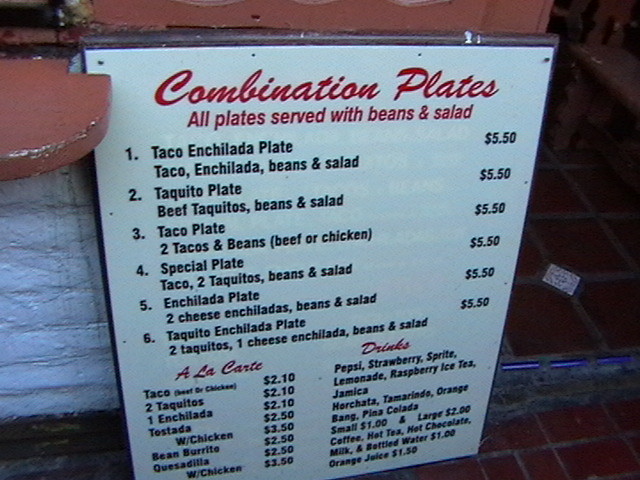In this photo, a large, prominent sign is displayed, leaning against a building. The sign features a white background with bold, cursive red letters at the top that read "Combination Plates." Below this heading, a subtext in red informs customers that "All plates served with beans and salad." The menu is then listed with numbered items and their prices:

1. **Taco Enchilada Plate - $5.50**
2. **Taquito Plate - $5.50**
3. **Taco Plate - $5.50**
4. **Special Plate - $5.50**
5. **Enchilada Plate - $5.50**
6. **Taquito Enchilada Plate - $5.50**

Further down, another section titled "A la Carte" in red text includes individual items and their respective prices:

- **Taco** - $2.10
- **Two Taquitos** - $2.10
- **One Enchilada** - $2.10
- **Tostito with Chicken** - $2.50
- **Bean Burrito** - $2.10
- **Quesadilla with Chicken** - $2.50

In a third section, the word "Drinks" is highlighted in red text, followed by a list of beverages in black text offering:

- **Pepsi**
- **Strawberry**
- **Sprite**
- **Lemonade**
- **Raspberry Iced Tea**
- **Orange Drink**
- **Piña Colada**
  
Prices for drinks are clearly marked:

- **Small** - $1
- **Large** - $2

Additional drinks include:
- **Coffee**
- **Hot Tea**
- **Hot Chocolate**
- **Milk**
- **Bottled Water**
- **Orange Juice** for $1